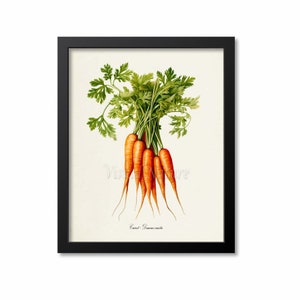This hand-painted artwork features a vivid cluster of carrots centrally positioned on a white background, framed within a thin, rectangular black frame that contrasts against the white wall it hangs on. The carrots, numbering around eight or nine, are depicted with a bright orange hue and subtle yellowing on the sides, tapering to very thin, fine points at their long roots. Each carrot is topped with multiple lush green leaves resembling cilantro, giving the impression they were freshly pulled from the ground. The green stalks are intricately detailed, enhancing the vibrant composition of the painting. Below the cluster of carrots, there's an illegible black cursive signature that adds a touch of authenticity to the artwork. This detailed and lively painting captures the essence of nature's bounty within its small, elegant frame.